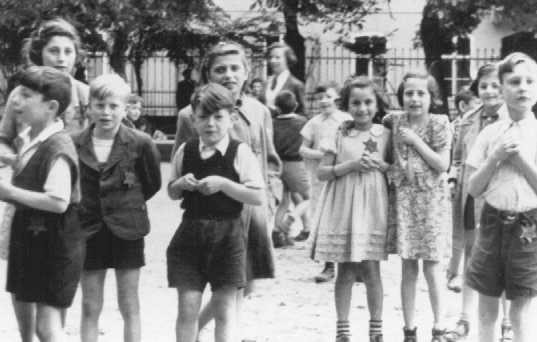This is a black-and-white photograph capturing a group of elementary school-aged children, likely from the 1950s or 60s. The children are posing in an open courtyard with a wrought-iron fence as a backdrop. The boys are dressed in short pants and short-sleeved button-up shirts, with some wearing sweater vests and one in a blazer. The girls sport dresses that generally reach their knees, some of which feature floral designs. Notably, several children have Stars of David pinned to their clothing, indicating they may be Jewish children in Nazi Germany. Both boys and girls display a mix of hair colors and styles, with boys having short hair and girls wearing theirs long and wavy. Among the children stand a couple of parents and a few older women, possibly in their late teens, with one adult supervising, suggesting a school recess or outdoor gathering. The children are mostly looking forward, directly at the camera, which captures a poignant and historically significant scene.